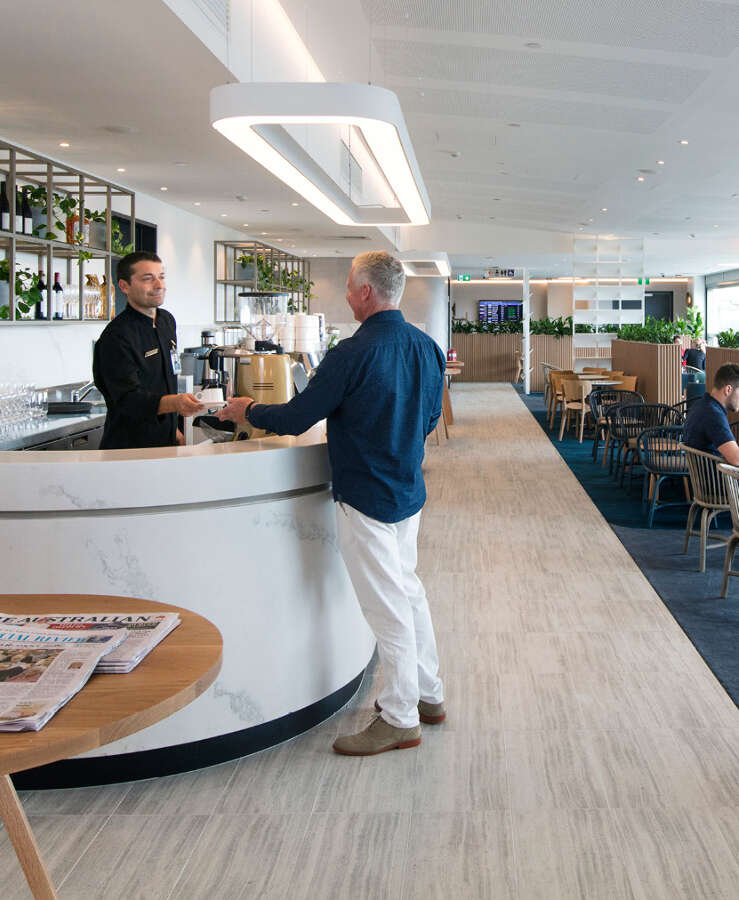The photograph captures the inviting atmosphere of a cozy establishment that appears to be a bar or lounge with a health-focused twist. On the left side, a long bar with a white countertop is a focal point, featuring an array of pitchers, glasses, and coffee-making machines. Behind the bar stands a smiling server, dressed in a black uniform adorned with a silver accent and a name tag, handing a coffee cup to a customer. The customer, an older man with gray hair, is positioned centrally in the scene, wearing a dark blue long sleeve shirt, white pants, and grey and brown shoes. Both men are bathed in the gentle light of a white chandelier hanging overhead.

Wooden shelves filled with various green plants line the back wall behind the counter, adding a touch of nature to the contemporary setting. To the right side of the room, a mix of round and square tables with assorted chairs accommodates other patrons, who can be seen enjoying their drinks and conversations. A television mounted in the background provides additional ambiance to the lively setting. In the foreground, a small wooden table prominently displays two different newspapers, inviting patrons to catch up on the latest news. The detailed depiction creates a warm, communal, and vibrant snapshot of everyday life within this bustling venue.